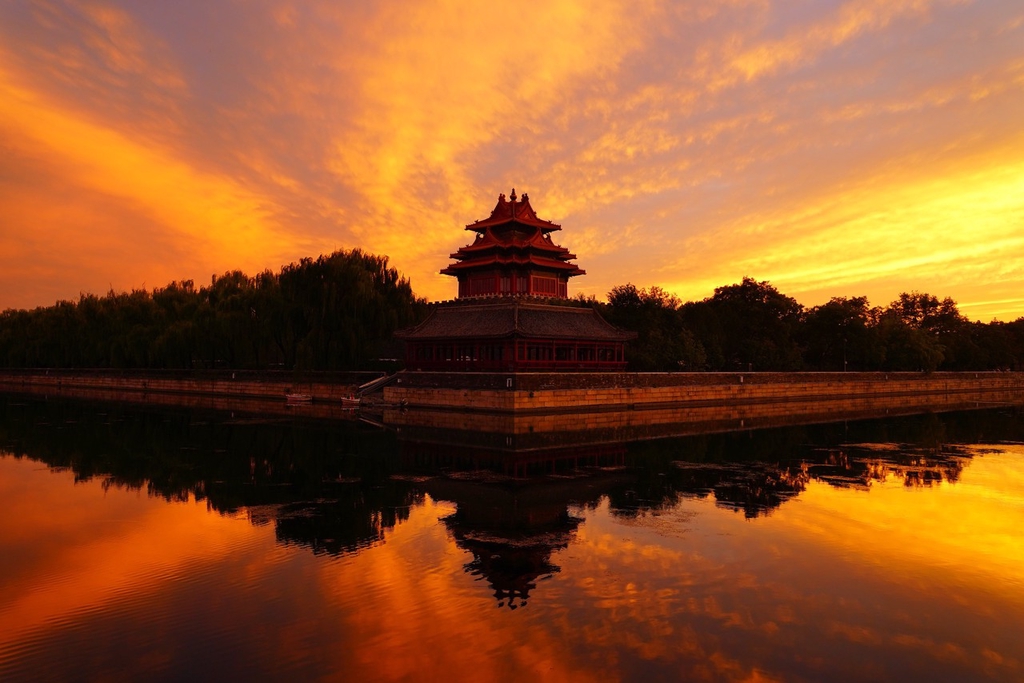The photograph captures an enchanting oriental-style temple centered within a serene scene, surrounded by a protective body of water, likely a moat. The temple, with its square base and towering central structure crowned by three tiers of roofing, stands majestically behind a stone and brick wall that separates it from the water. Lush trees envelop the temple, emphasizing its isolation and tranquility. The sun is setting, painting the sky in a gradient of orange hues, with deeper shades on the left transitioning to brighter tones on the right, and traces of dark blue. This vibrant coloration of the sky, along with the silhouetted clouds tinged with orange, is beautifully mirrored in the calm waters below, further enhancing the ethereal atmosphere of the scene.